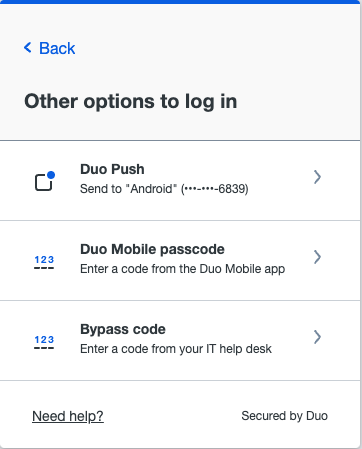**Caption:**

A detailed screenshot showcasing alternative login methods, likely from a mobile device interface. The background is predominantly white, with black and blue text providing instructions and options.

At the top, blue text with a bold "Back" and a "<" symbol allows navigation to the previous page. Below, a black heading reads, "Other options to log in," followed by three distinct login options presented in boxes.

1. **Duo Push**: Displayed in bold black text, featuring an icon of a square box with a blue circle in the top right corner. The text instructs, "Send to ‘Android ***-***-6839’," with a gray arrow indicating further action.
   
2. **Duo Mobile Passcode**: Depicted with an icon showing the numbers "123" separated by dashes. The instruction reads, "Enter a code from the Duo Mobile app."
   
3. **Bypass Code**: Illustrated with the same "123" icon. The accompanying text prompts, "Enter a code from your IT helpdesk," also followed by a gray arrow for additional steps.

At the bottom, the text "Need help?" appears, followed by "Secured by Duo," highlighting security features.